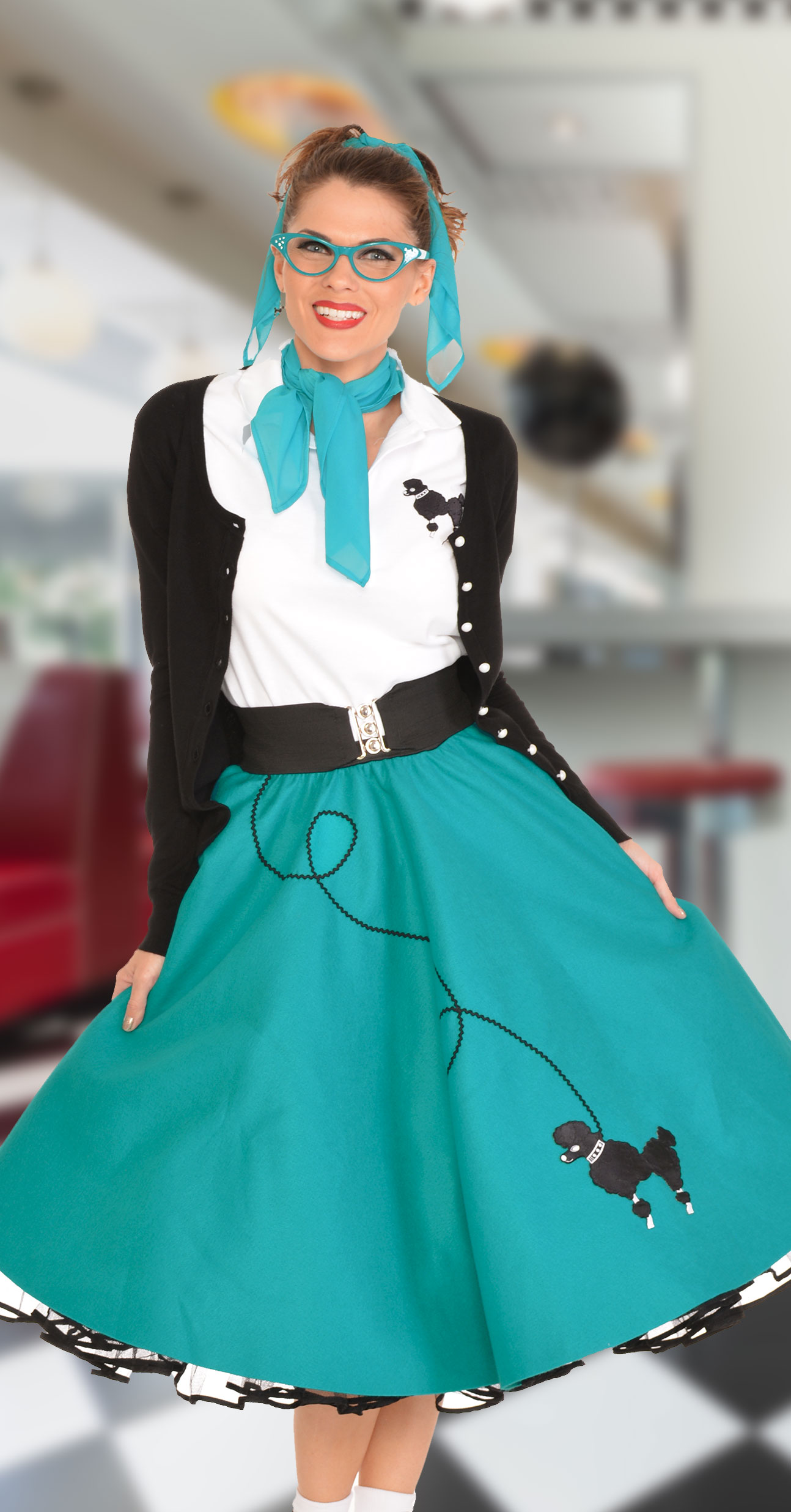In this lively and nostalgic image, a young woman is captured in a vibrant 1950s-themed outfit, standing confidently in a classic diner setting adorned with a silver counter, red stools, black ceiling fan, and recessed lights. She is dressed in a teal poodle skirt featuring a detailed black poodle emblem with a white collar and a leash that artistically twines up towards her black belt. Her outfit is completed with a black cardigan sweater adorned with white buttons over a white blouse that also sports a black poodle emblem on the right breast. A teal neckerchief and a matching teal bow in her hair add a touch of flair, coordinating with her teal horn-rimmed glasses. She wears bright red lipstick and bobby socks with black and white frills underneath, holding out the sides of her skirt to showcase its full flair. Her joyful smile and poised stance suggest she's ready for a lively jitterbug, embodying the essence of the 1950s. The checkered tile floor and booths in the background further enhance the retro atmosphere, encapsulating a perfect slice of mid-century Americana.